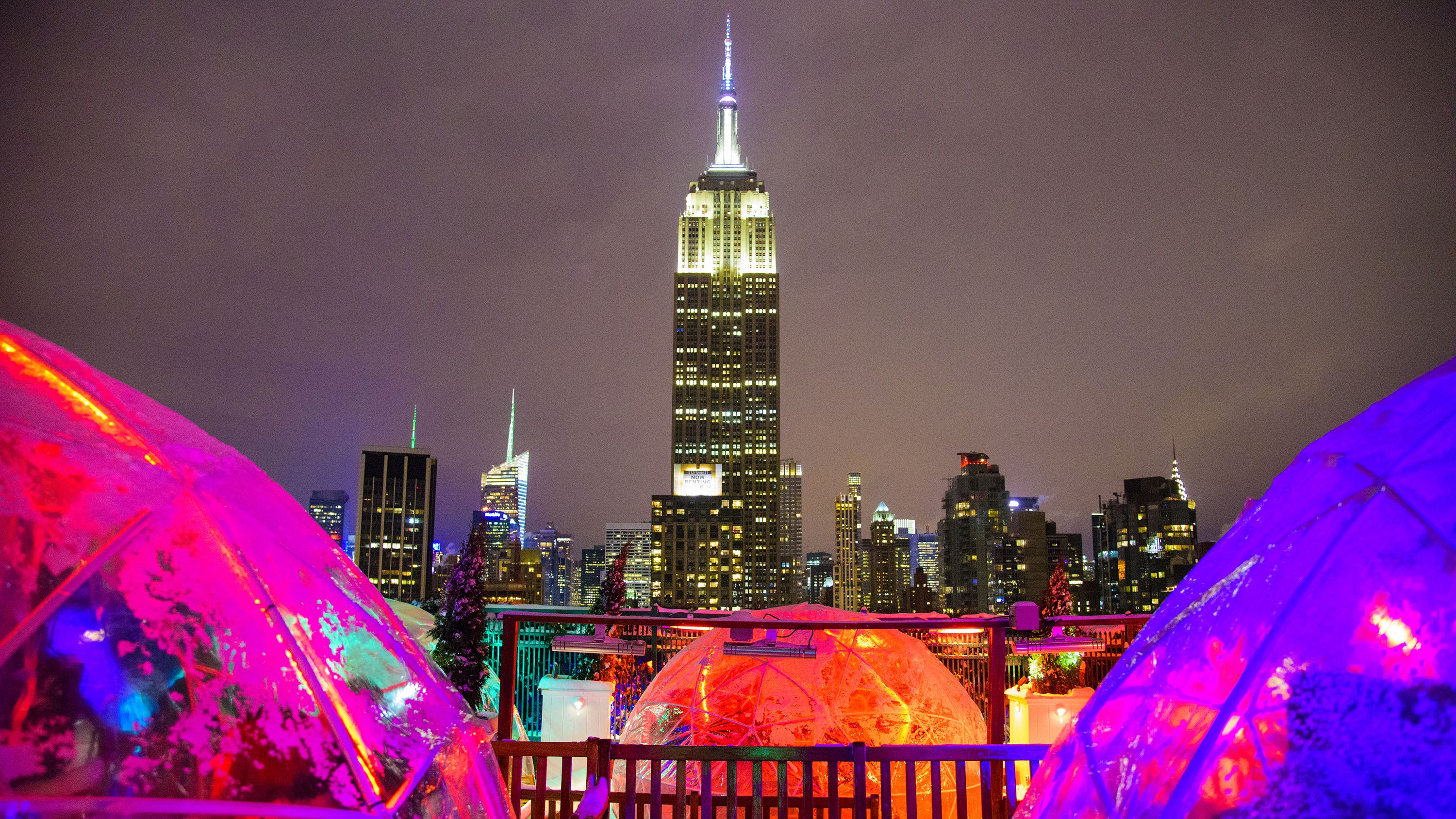The image showcases a vibrant city skyline at night, dominated by a towering skyscraper adorned with light greenish-yellow illumination and crowned with a prominent steeple. Surrounding this central skyscraper are various other buildings that, although impressive, are comparatively shorter. In the foreground, three large, illuminated domes add a splash of color; each dome shines in a different hue – one pink, one orange, and one purple. These domes are separated from the rest of the scenery by a wooden railing, behind which a third dome is partially visible. Above, a gray and cloudy sky blankets the city, enhancing the night-time ambiance. The city’s skyline stretches into the distant background, completing this detailed urban scene.